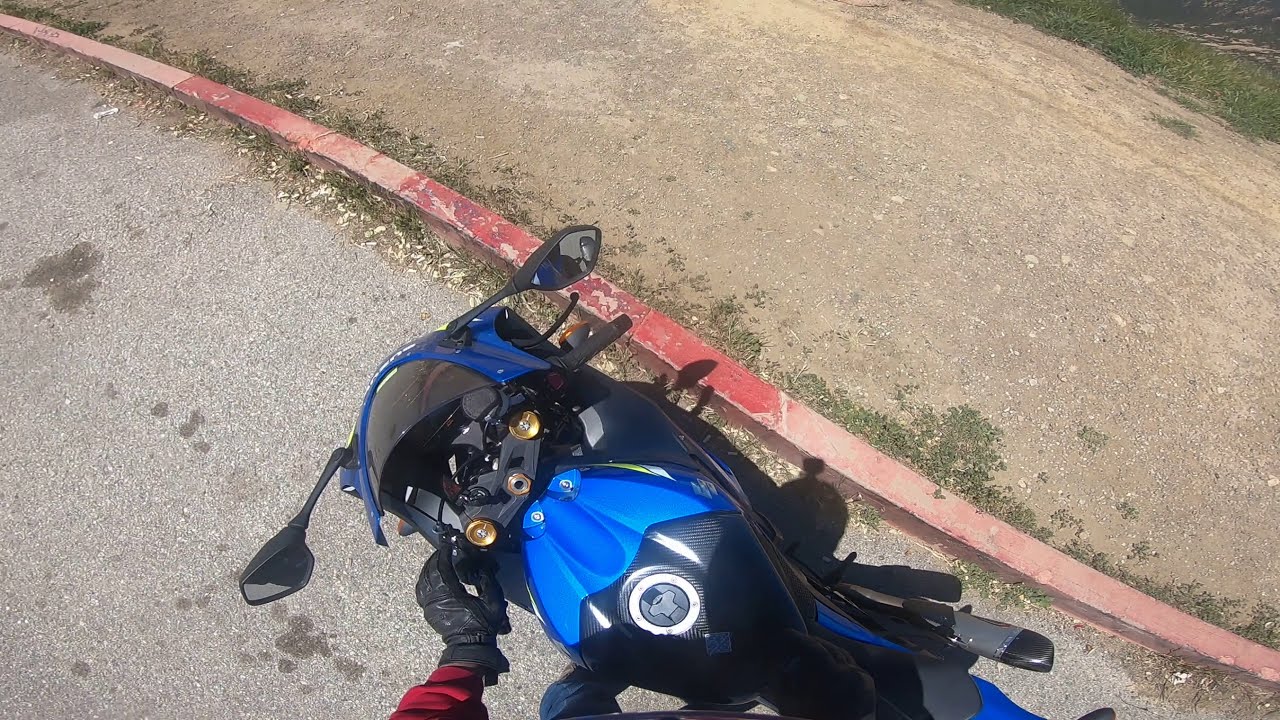The image is a landscape-oriented color photograph, captured as a freeze-frame from a GoPro video mounted on a rider's helmet. The point-of-view shot focuses on a blue motorcycle with a carbon fiber gas tank and black controls, parked beside a red curb, suggesting a no-parking zone. The motorbike features a low blue windshield and two black rear-view mirrors. The rider's left arm is partially visible, adorned in a long-sleeve red shirt and a black leather glove gripping the handlebars. The surrounding area includes a gravel path to the left and a paved path with a patch of grass in the upper right corner. The overall scene exemplifies representational realism, giving a detailed and lifelike perspective from the rider's view.